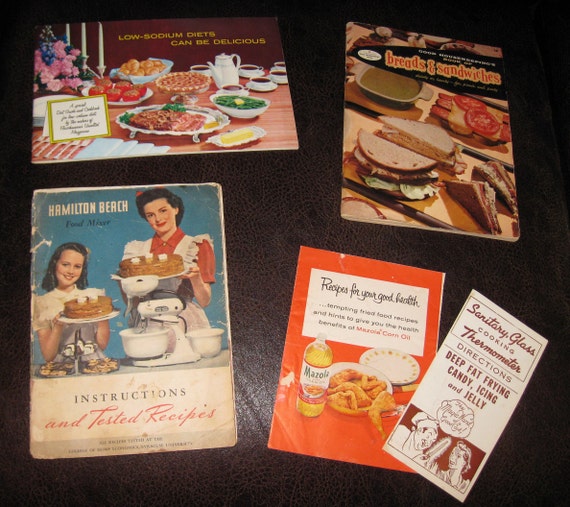The image shows an assortment of vintage cooking pamphlets and booklets placed on a shiny black or dark brown leather-like surface. At the top left, there is a colorful pamphlet featuring various plates of food on a wooden table, including ribs, pie, beans, butter, yams, rolls, and cups of tea or coffee served in white cups. This pamphlet is titled "Low-Sodium Diets Can Be Delicious," suggesting creative and tasty low-sodium recipes.

To the right, there's another booklet titled "Breads and Sandwiches" with visuals of various sandwiches filled with ingredients like cheese, ham, lettuce, and tomatoes. 

At the bottom left, an aged, tattered booklet labeled "Instructions and Tested Recipes" from the Hamilton Beach Food Mixer features an image of a woman wearing a red shirt and white apron, holding a cake, with a girl beside her also holding a smaller cake. The mixer can be seen in front of them.

At the bottom right, two more pamphlets are visible. One, colored orange and white, is titled "Recipes for Your Good Health" and includes tempting fried food recipes, emphasizing the health benefits of using mozzella corn oil. The other white pamphlet titled "Sanitary Glass Cooking Thermometer Directions" covers topics like deep fat frying, candy making, icing, and jelly, and features an image of a man and a woman. 

Collectively, these items reflect a nostalgic theme of culinary guides dedicated to various aspects of cooking and healthy eating.